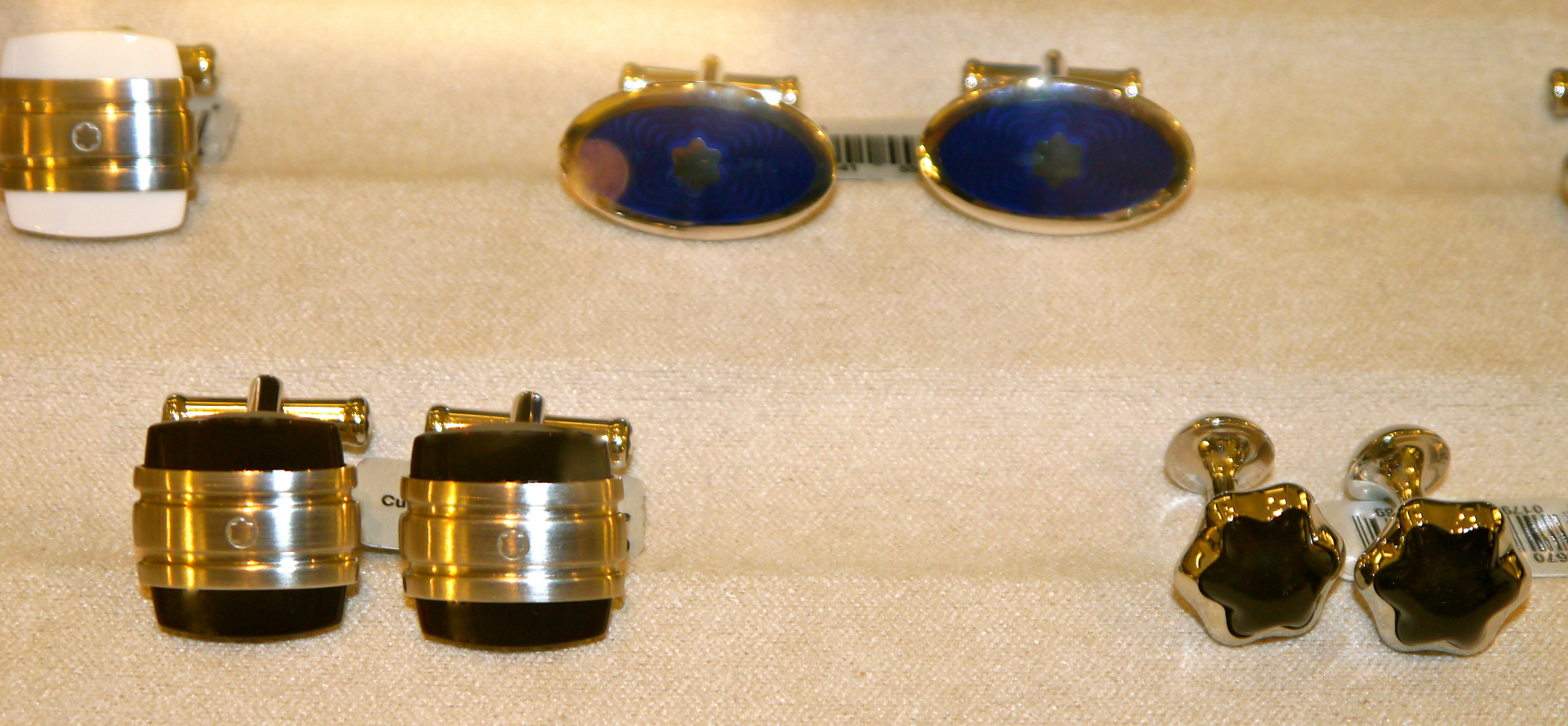This photograph features a close-up collection of four pairs of cufflinks arranged on a light brown, fine cloth background. In the bottom right, a pair of golden hexagon-shaped cufflinks is adorned with a bold black six-pointed star at their center. In the bottom left corner, a second pair of black square cufflinks features a distinctive golden band through their center. In the background, an elegant pair of oval-shaped cufflinks showcases a dark blue and black swirl pattern with a six-pointed star encased in a golden border. In the top left corner, partially visible, is a single white cufflink with a matching golden band similar to the black square pair below. The overall composition highlights intricate designs and a blend of gold, black, and blue tones, emphasizing both the cufflinks' craftsmanship and luxurious appearance.